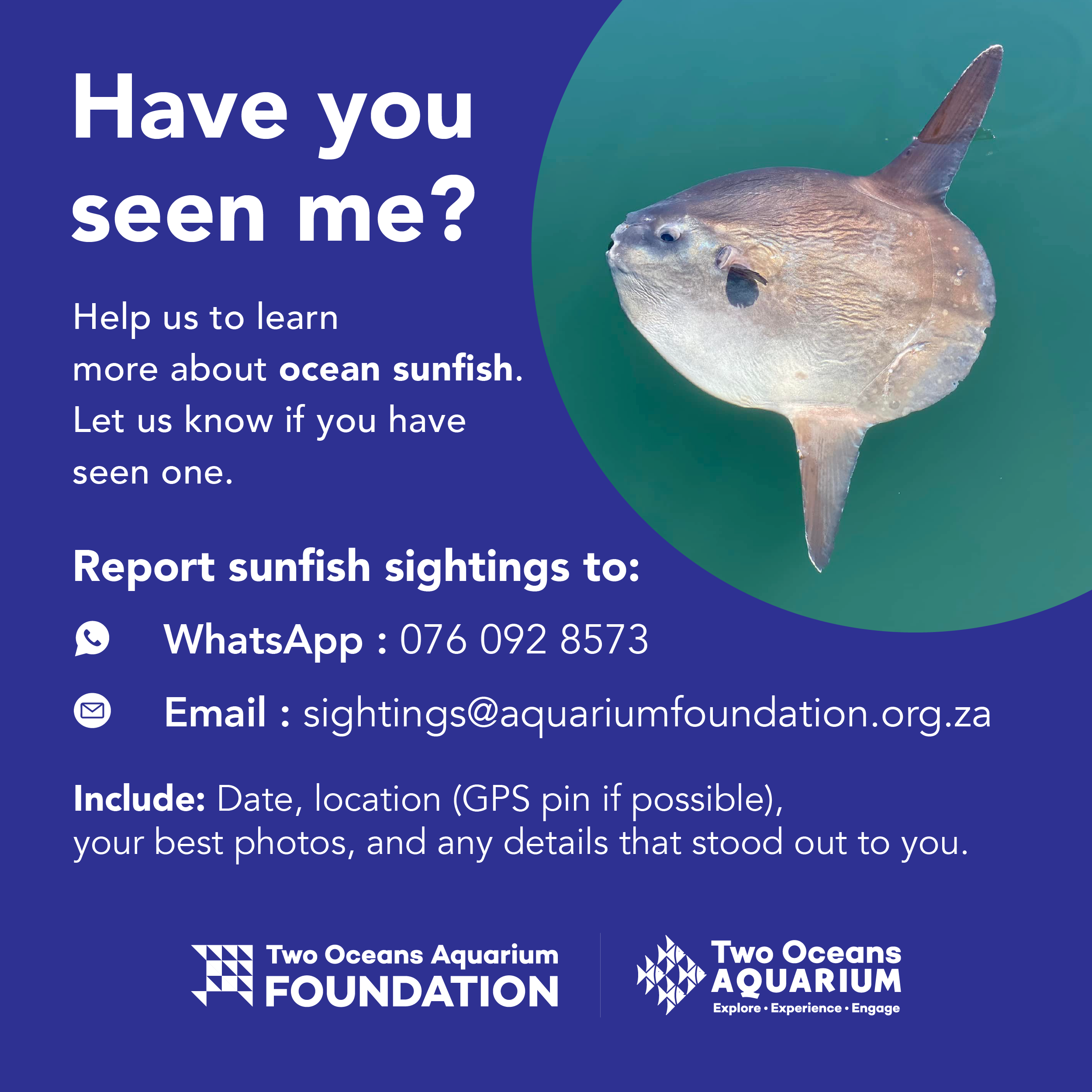This image is an awareness flyer predominantly in dark blue with a hint of teal, designed to gather information about ocean sunfish sightings. The flyer features a gray sunfish with a dorsal fin and a bottom fin, set within a lighter sea green circular section at the top right corner. Accompanied by the bold white text, it reads: "Have you seen me? Help us learn more about ocean sunfish. Let us know if you have seen one." Below, it requests that sightings be reported via WhatsApp at 076-092-8573 or email at sightings@aquariumfoundation.org.za, and asks for the date, location (including GPS pin if possible), best photos, and any notable details in the report. At the bottom, the flyer displays two logos: one for Two Oceans Aquarium Foundation and another reading "Two Oceans Aquarium: Explore, Experience, Engage."